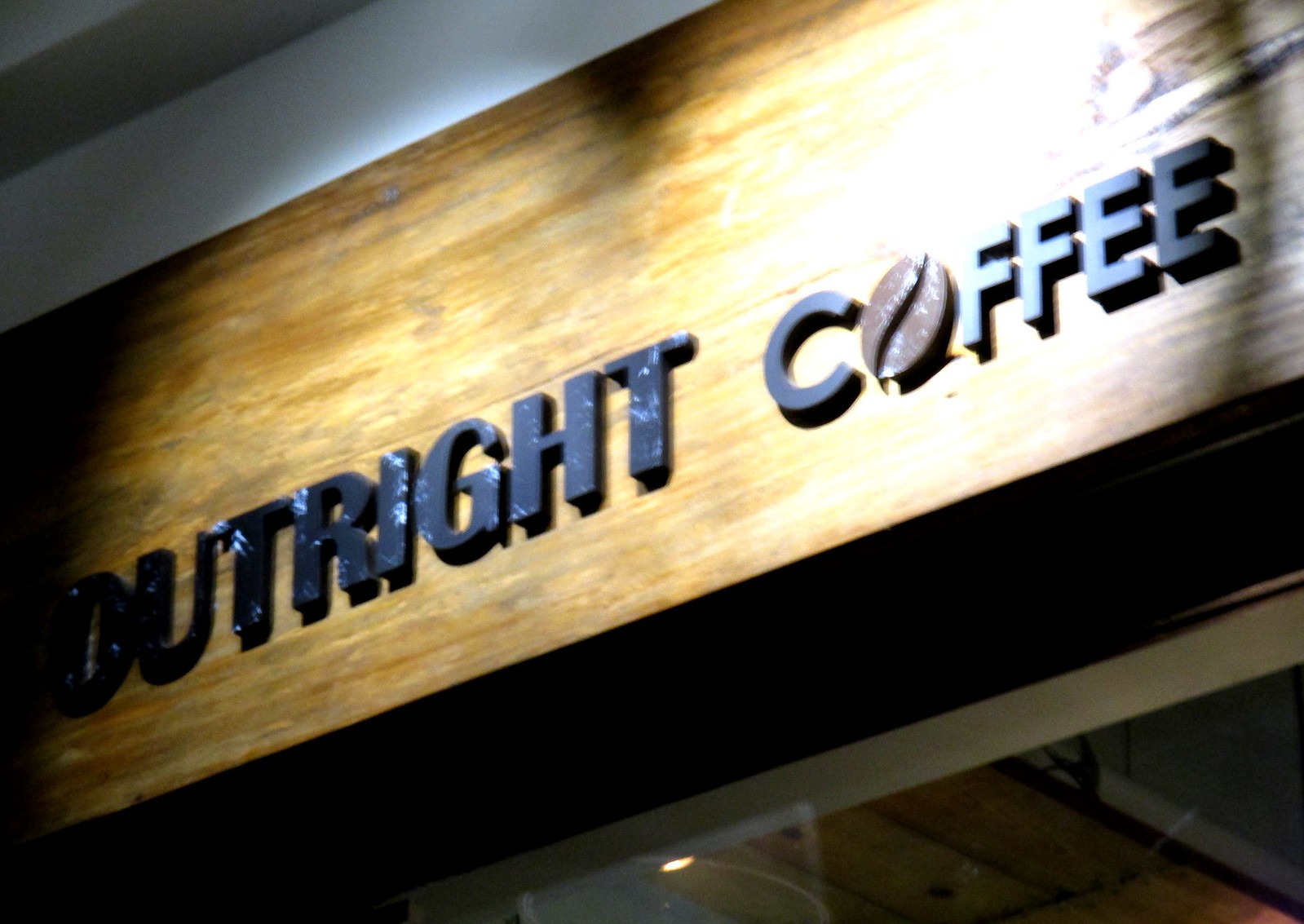This photograph features the commercial signage for a business named "Outright Coffee," prominently displayed on a wooden facade above the shop’s entrance. The wooden sign, bathed in light, reveals the shop name in uppercase letters. While the letters are mostly black, they appear marbled with white specks that add a distinct texture. The 'O' in "Coffee" is creatively replaced by a brown coffee bean icon. The image captures the sign at a slight angle, ascending from the lower left to the upper right, with parts of the storefront, including the glass entryway and dimly lit interior lights, visible beneath. The overall ambiance of the picture is accentuated by the lights shining on the sign, making it a focal point against the darker surrounding elements.